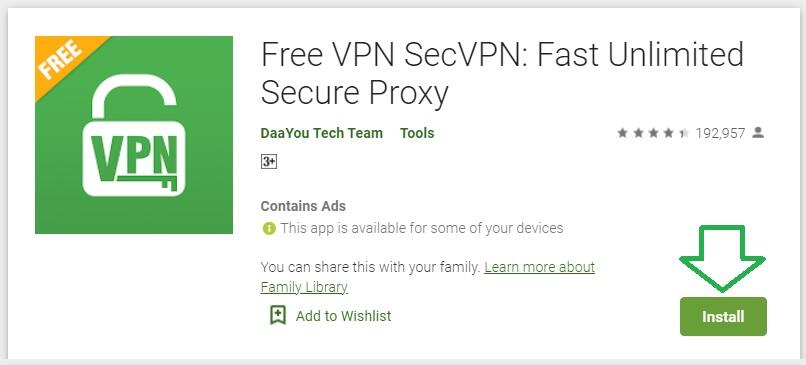This screenshot captures a downloadable app interface on a device screen. The main background is white with a prominent green box. Within the green box, there's a solid green square, and in one of its corners, a triangle displays the word "Free" in white and yellow. The app icon prominently features a green key and a white lock beneath the letters "VPN," also in green.

To the left of the green box, detailed text describes the app as "Free VPN - SecVPN: Fast, Unlimited, Secure Proxy," followed by the developer's name, "Dayutech Dream," written in green. The app holds a rating of 4.2 stars, based on feedback from 192,957 users. It is rated suitable for ages three and up. Additional information indicates that the app contains ads and is available on some of your devices. It also mentions the possibility of sharing the app within a family group and learning about the Family Library.

At the bottom right, there are buttons for sharing the app and an option to add it to a waitlist. An arrow pointing down leads to the "Install" button, which is written in white.